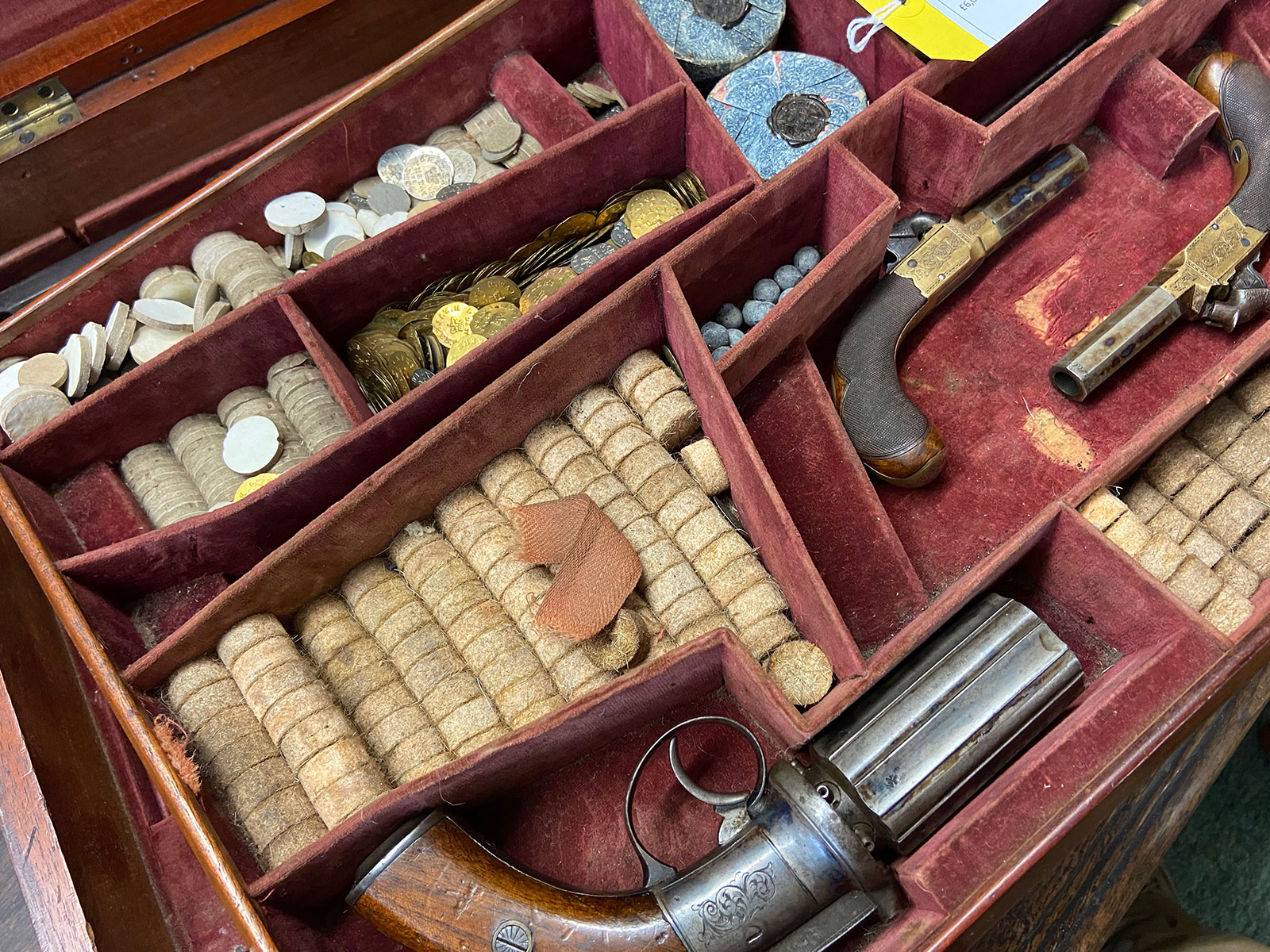The photograph captures the interior of an antique wooden storage case, showcasing a well-preserved collection of old artifacts. The case, positioned at an angle, opens to reveal a rich, burgundy velvet lining, though the fabric is worn and faded in several places, exposing the underlying brown wood. Gold hinges on the lid suggest a touch of elegance and age.

Dominating the center of the case are several guns, each nestled neatly within their designated compartments. At the bottom, a six-barreled pistol with a wooden handle stands out, reminiscent of a Gatling gun but in a handheld form. To the right of this, two slender, single-shot pistols with cylindrical barrels and flintlock caps are arranged side by side, their metal parts showing signs of rust, indicating their antique nature.

Scattered throughout the compartments are various circular objects. Some sections contain what appear to be old coins, with one section showcasing shiny gold coins and another, duller, silver ones. Other compartments hold rows of small, cylindrical disks made of fabric or pressed material, resembling cork or pellets, possibly used for gambling or as imitation coins. Among these artifacts, a hint of blueish metal balls, suggesting old bullets, contrasts with the earthy tones of the case's contents.

Overall, this intricate case is a treasure trove of historical items, possibly a gambler's toolkit, filled with relics that paint a vivid picture of a bygone era.